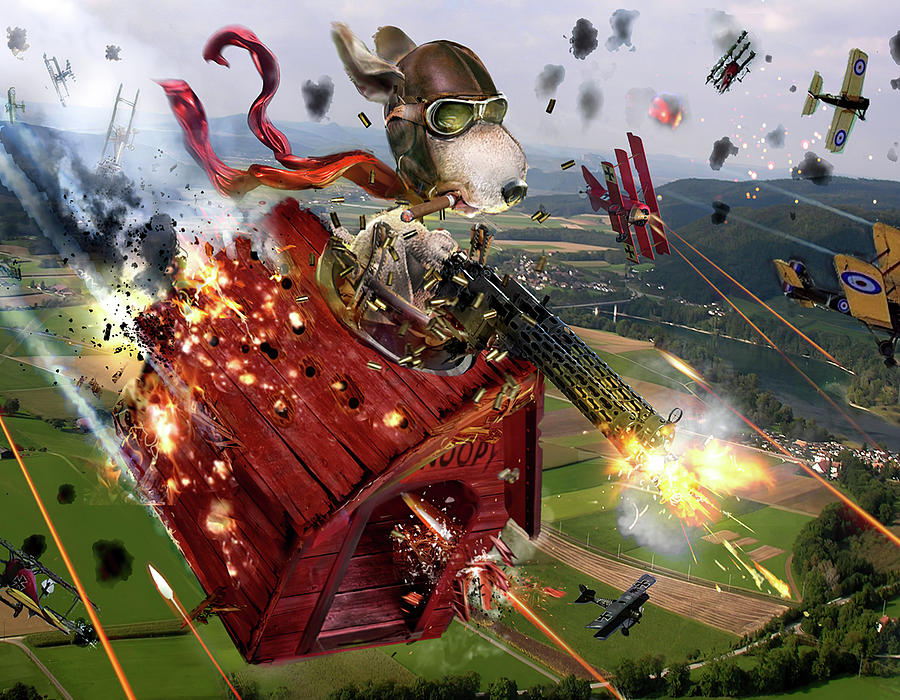In this vibrant, horizontal rectangular image, Snoopy, the iconic beagle from the Peanuts comic strip, is depicted as a World War II flying ace. He is boldly piloting his red doghouse through the sky, which is riddled with bullet holes and emitting smoke. Snoopy is wearing a dark brown leather pilot’s helmet, goggles, and a red scarf that flies dramatically behind him, adding to his heroic demeanor. A cigar juts from his mouth as he shoots a machine gun attached to his doghouse, aiming downward toward unseen targets below. 

The doghouse itself bears numerous bullet holes with flames and smoke escaping from the damage, illustrating the intensity of the aerial battle. Surrounding Snoopy are several airplanes of various colors, including red, gold, and gray, each similarly engaged in fierce combat. Parachutes and targets are scattered in the sky, adding to the chaotic battle scene. Beneath the doghouse lies a lush, green field area, possibly a football field or an airport, dotted with trees and small houses. The background extends into rolling hills under a clear sky, framing this dynamic and whimsical air battle with a cartoonish charm. The entire scene captures the essence of a wartime dogfight, albeit with Snoopy's humorous and fantastical twist.